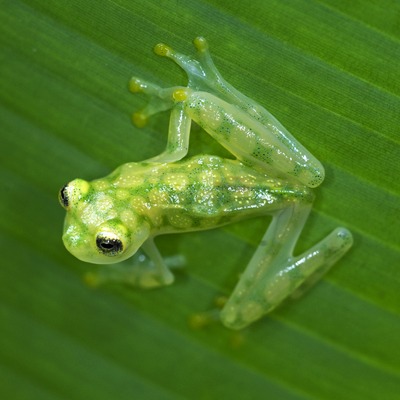This is a photograph of a tiny, bright green tree frog with a translucent, almost transparent appearance. The frog's delicate body features both pale green and bright yellow camouflage spots, and it has prominent black, oval-shaped eyes with horizontal pupils. The frog is viewed from above, positioned in the middle of the frame, sitting on a large striated leaf that appears dark green, possibly resembling a palm frond. Its legs are drawn up underneath it in a seated position, with its tiny feet displaying small yellow suction cups at the tips of its toes. The frog looks glossy and damp, seemingly poised to hop to the left.